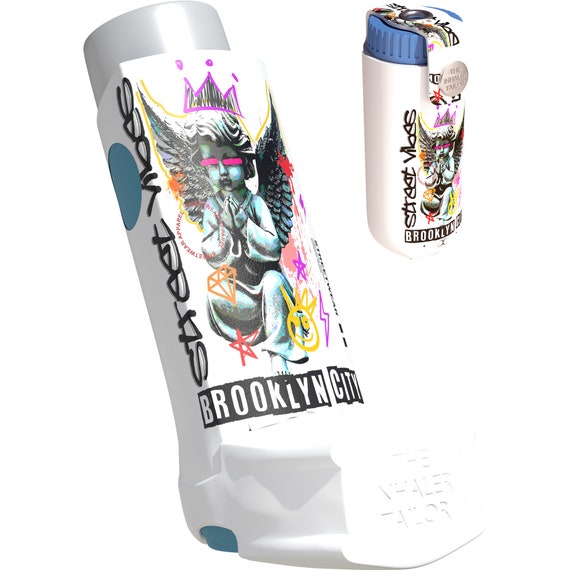The image features two digitally drawn asthma inhalers against a white background, both embellished with graffiti-style artwork. The larger inhaler is positioned to the left and has a gray, round top with a vertical rectangular body. This body is predominantly white with vibrant artwork depicting a child sitting with hands together, angel wings spread behind them, and a hand-drawn crown on top. Below this, text reads “Brooklyn City” and vertically, it says "Street of Vibes". Additionally, there's a subtle, white all-caps print near the bottom that reads "The Inhaler Tailor". 

To the upper right is the smaller inhaler with a blue top. It mirrors the design of the larger one, also featuring the child as an angel, the graffiti text "Street Vibes" and "Brooklyn City". Both inhalers are decorated with multiple logos, including a diamond, a star, a smiley face, and a lightning bolt.